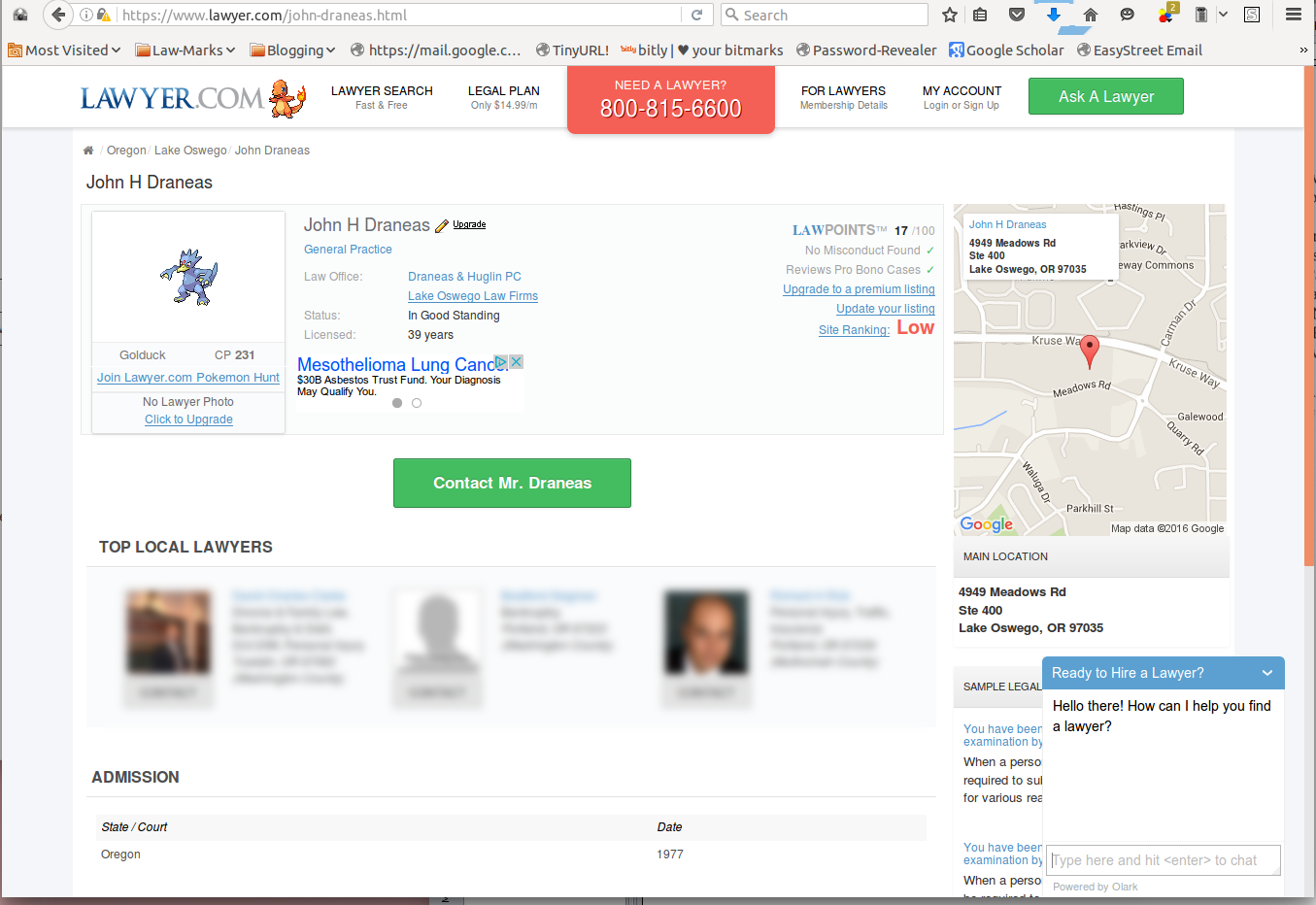The image depicts a webpage from the browser opened to Lawyer.com, specifically on a search page for lawyers. The top section highlights a promotion for a legal plan costing $14.99 per month. Below this is a prominent red rectangle featuring a white linear text promoting the service, along with a helpline number: 800-815-6600. There are also links for membership details, and options for logging in or signing up.

On the left-hand side, there is a green button labeled "Ask a Lawyer." Below this button, the page displays specific information about a local lawyer named John H. Draneas located in Lake Oswego, Oregon. His profile contains his name and a section indicating his status, association with Dreyas and Higgins PC law firm, and that he has been licensed and in good standing for 39 years. The profile hints at his specialties and mentions conditions related to methicillinoma and lung cancer, associating them with a $30 billion asbestos trust fund, suggesting potential clients might qualify for compensation.

The page also appears to offer a feature to upgrade the lawyer's profile picture and edit details, pointing out it is editable and contactable.

This detailed description gives a comprehensive understanding of what is shown on the webpage.